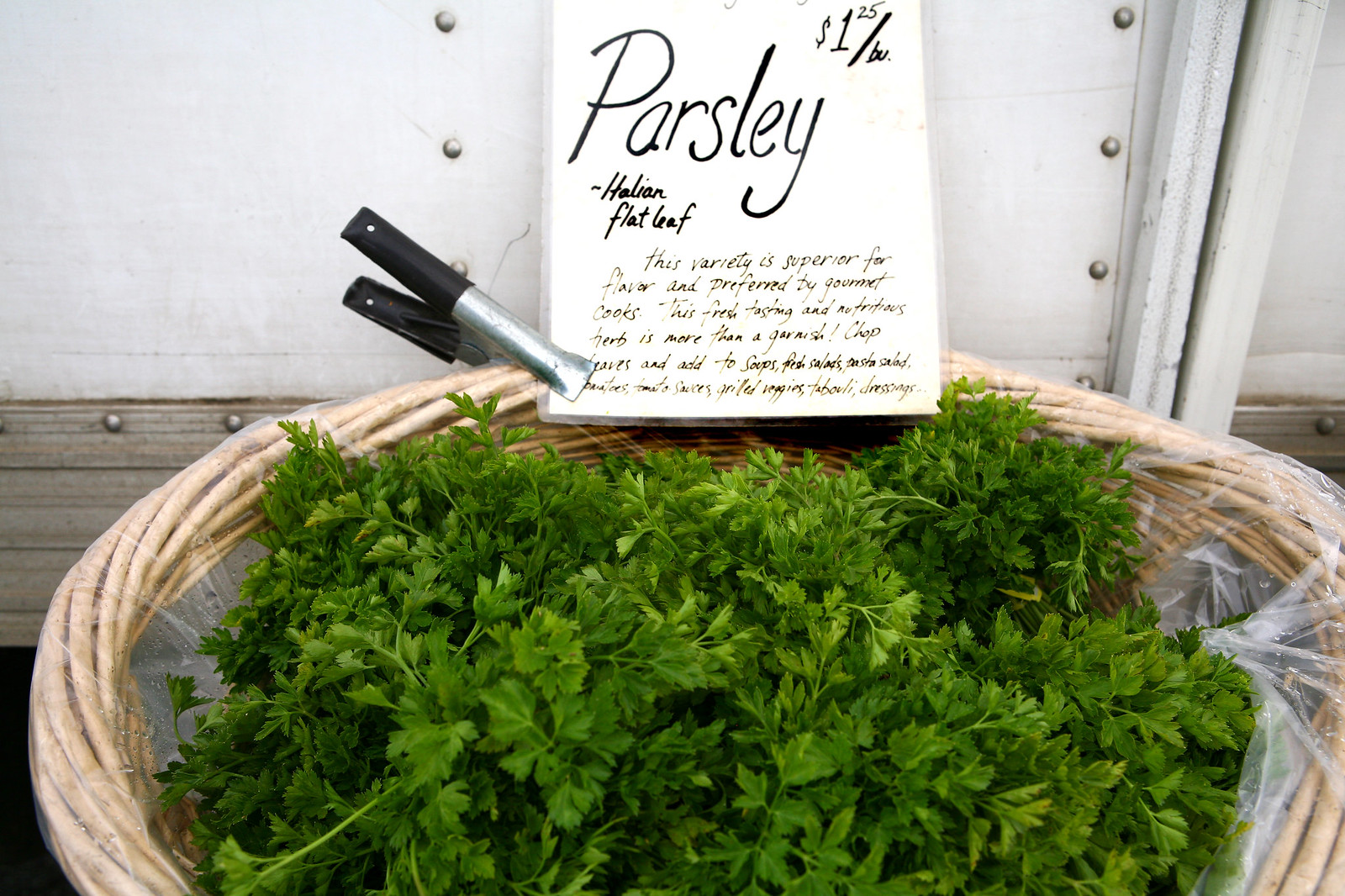A meticulously detailed photograph depicts a wicker basket, lined with a clear plastic bag, brimming with vibrant green Italian flat-leaf parsley. The basket sits in what appears to be an open market, with a distinctive metal clamp—silver with black handles—securing a white piece of paper to its edge. The paper label reads prominently in black marker: "Parsley, $1.25 per bundle," and "Italian Flat Leaf." Below this, a detailed description highlights the herb's culinary superiority, cherished by gourmet cooks for its flavor. The text underscores that parsley, fresh and nutritious, transcends mere garnish status, suggesting it be chopped and added to soups, salads, pasta salads, tomato sauces, grilled vegetables, tabbouleh, and dressings. The backdrop reveals a white metal wall with visible studs and bolts, and a weathered wooden board at its base, adding a rustic charm to the market scene.